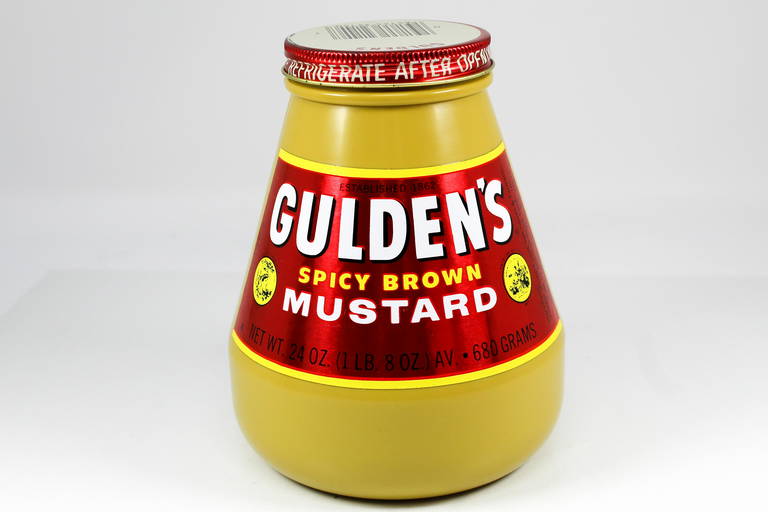This close-up image features a distinctive bottle of spicy brown mustard by Gulden's, prominently displayed in a lightbox. The plastic bottle has a wide, rounded base that tapers into a narrower neck, almost teardrop-shaped but flat at the top, resulting in a triangular appearance. The vibrant, deep yellow bottle is accentuated by a shiny red label, which has white text spelling out "GULDEN'S." Beneath, in bright yellow text, the label reads "SPICY BROWN," followed by "MUSTARD" in white. The bottle holds 24 ounces (680 grams) of the mustard and is sealed with a metal screw-on cap. The cap is red with white text instructing to "REFRIGERATE AFTER OPENING." In the backdrop, the subtle outline of the lightbox's white walls enhances the focus on the bottle's design and labeling.